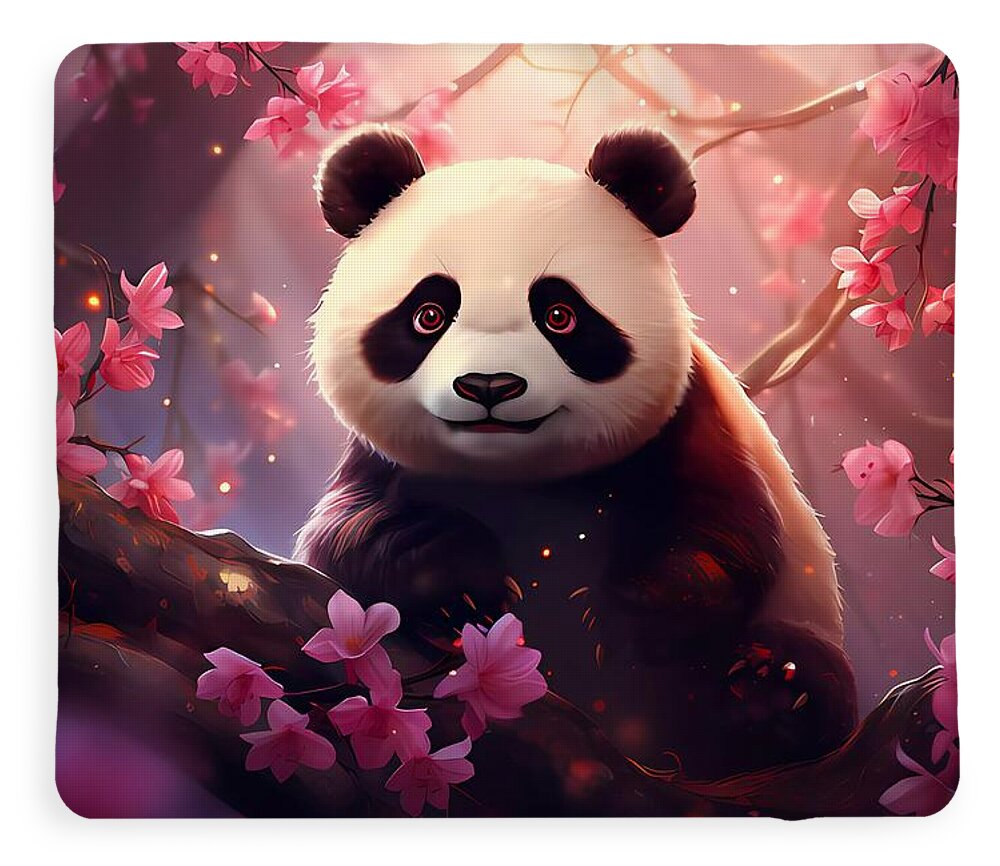This vibrant digital illustration depicts a charming, comical panda engaging the viewer with its large, expressive brown eyes and a sweet, smiling expression. The panda, featuring distinctive black ears, a black nose, and striking black-and-white fur, appears hunched over slightly, as if about to grasp a tree branch adorned with delicate cherry blossoms. Amidst the misty, blurred background, which creates an ethereal atmosphere, pink flowers and floating white specks surround the panda, enhancing the whimsical nature of the scene. The scene is illuminated by a soft, yellowish glow from above, resembling a gentle spotlight, further highlighting the panda's endearing presence. Its sharp claws are visible, adding a contrast to its otherwise cuddly appearance. The overall setting, with scattered cherry blossoms and mist, evokes a dreamlike, serene ambiance.